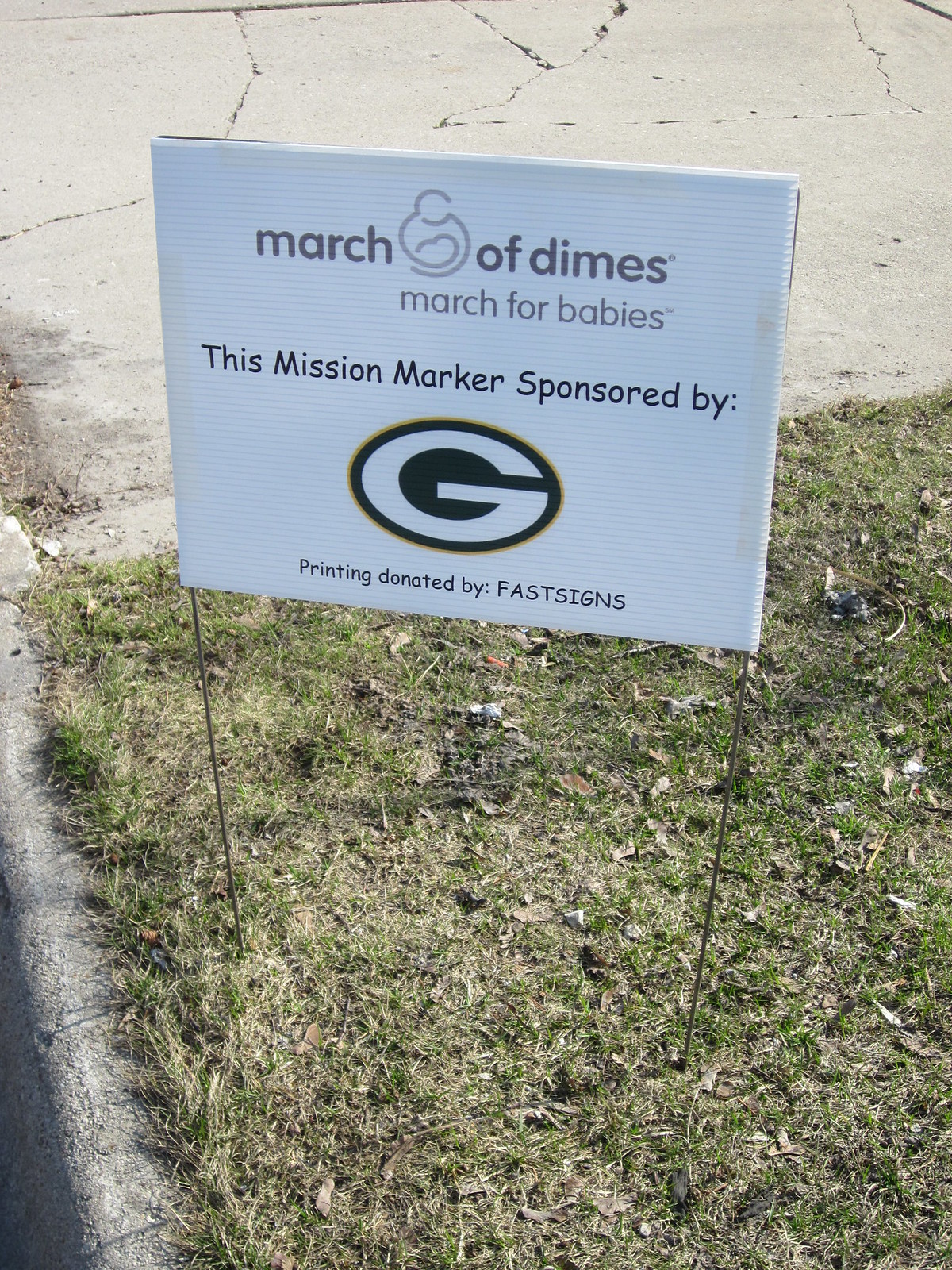The image displays a yard sign staked into a dry, somewhat patchy lawn with many dead leaves scattered about. The white plastic or hard paper sign, resembling those typically used for political campaigns, prominently features the text "March of Dimes, March for Babies." Beneath this, it states, "This Mission Marker Sponsored by," followed by the Green Bay Packers logo—a green oval with a white "G" and a gold border. Further down, the sign acknowledges, "Printing Donated by Fast Signs." The background includes a cracked concrete driveway or sidewalk, adding a subtle yet noticeable detail to the setting. The entire scene appears to be placed in the front yard of someone's home.